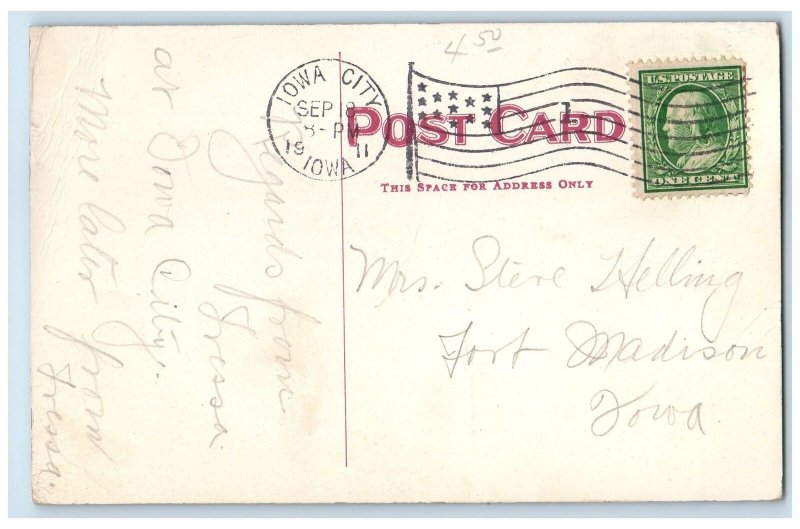This is a photograph of a vintage postcard with a faint blue outline, resting on a white background tinged with streaks of brown dirt and wear. The postcard features an array of distinctive marks and inscriptions. In the top left corner, there is a green, square U.S. postage stamp with the denomination of one cent, which has been partially obscured by a black American flag postmark. To the right of these elements, another stamp, in pink, reads "Postcard, this space for address only." 

Additionally, there's a circular postmark to the left that reads "Iowa City, September 8th, 8 PM, 1911, Iowa." Above these stamps, "450" is hand-written on the right side. The recipient's address is inscribed at the bottom right, reading "Mrs. Slane Helling, Fort Madison, Iowa."

On the left side of the postcard, there is a vertically oriented, handwritten note in cursive, composed of around four short lines, which is challenging to decipher. Part of the inscription seems to include names or words like "Rinaldo," "love," "Srisa," "our diva," and "Stresa." Another part of the note appears to address the recipient with words directed to “Miss Sleeve Alling.” The overall appearance of the postcard suggests it is both old and well-traveled, with the text and markings contributing to its rich, historical character.